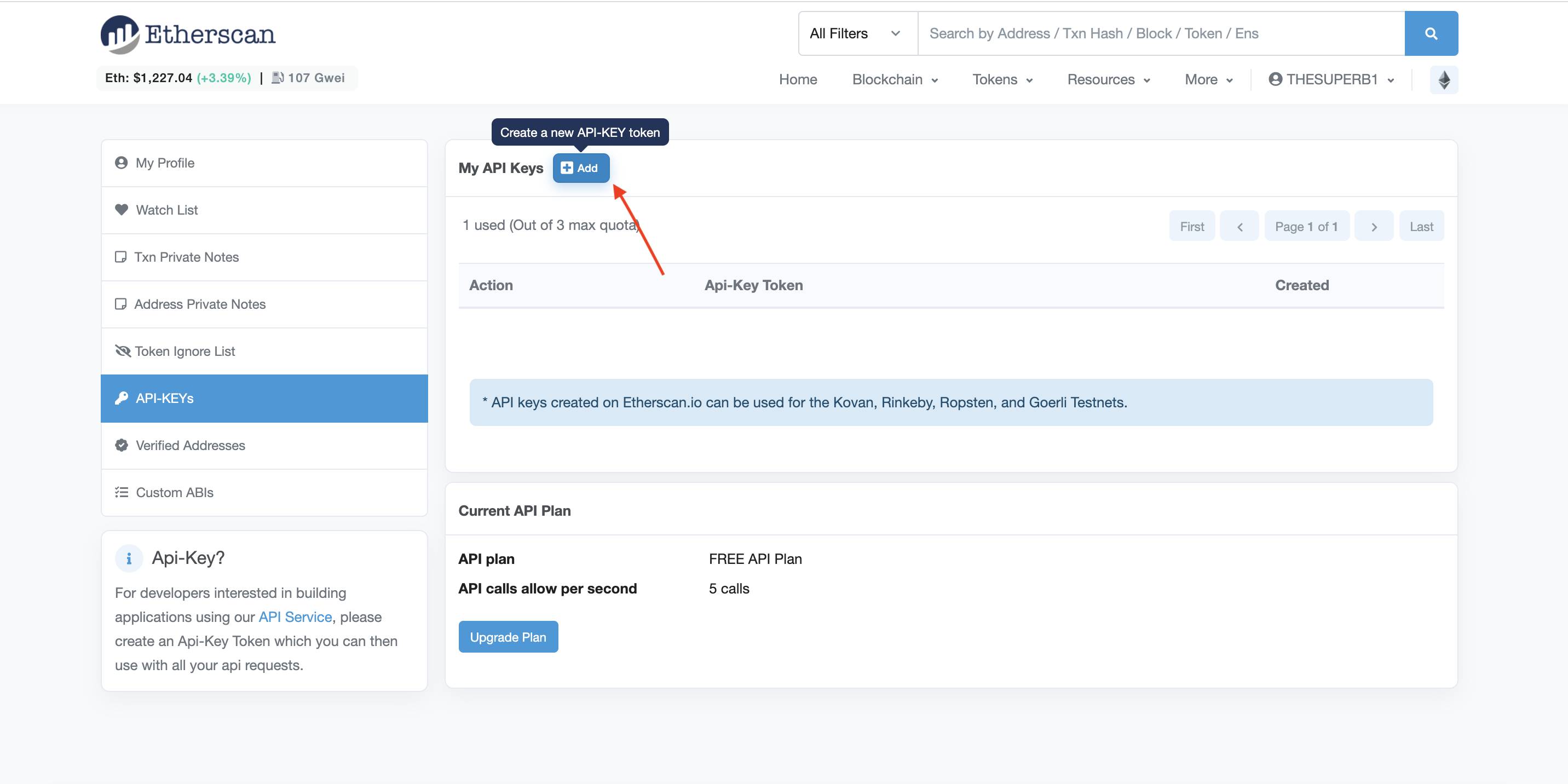A detailed, cleaned-up caption for the described image:

---

This screenshot displays the EtherScan website interface. In the top left corner, there is a small circular icon featuring blue, gray, and white colors. Directly beneath the icon, the current price of Ethereum is shown as "ETH $1,227.04" with a percentage change in green next to it, marked as "3.39%". 

To the right of this section, a search bar is available for users to search by address, TX (transaction), hash, block, token, or ENS, accompanied by a blue search button. The top navigation bar includes options labeled "Home," "Blockchain," "Tokens," "Resources," and a dropdown menu labeled "More."

There is also a blue button labeled "Create a New API Key Token." The website's background is predominantly white with black text, and some of the text is highlighted in either light blue or darker blue.

At the bottom section of the screen, the current API plan is detailed: "Current API Plan: Free API Plan." Users are informed that the free plan allows for five API calls per second and there is an option to "Upgrade Plan" in blue.

The left-hand sidebar contains several options: "My Profile," "Watch List," "TX and Private Notes," "Address Private Notes," "Token Ignore List," "API Keys," "Verified Addresses," and "Custom ABI's."

---

This description provides a comprehensive and clear depiction of the contents and layout of the EtherScan website as captured in the screenshot.